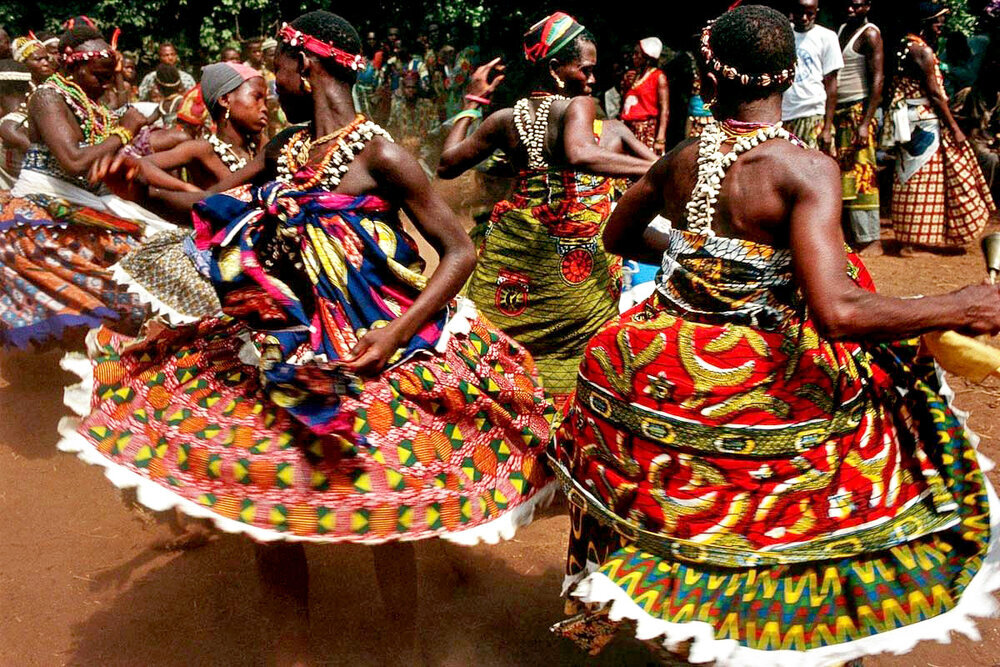The photograph captures a vibrant scene of African women dancing outdoors during the daytime on a dusty red dirt ground with some straw scattered about. The dancers, who are most likely African due to their dark brown skin and the cultural context, are adorned in ornately designed, bright, and colorful dresses that exude citrusy hues like orange and vibrant colors. Each woman’s dress has flowing skirts that depict vivid images of fruits, such as plantains, and is held up by straps made of white shells. The tops of their outfits are fashioned with bands of shells that tie around the front, crossing at the chest. They also wear a variety of head adornments, including colored headbands, caps, and beaded necklaces. The women have short-cropped hair, styled in a way that might seem masculine, enhancing the traditional aesthetic of their appearance. They dance with their arms extended to the sides, elbows bent, causing the fabric of their dresses to swirl around them in wide, expressive movements. In the background, the scene is set against a backdrop of green-leaved trees and other African onlookers who are watching the dance, enhancing the communal and festive atmosphere.